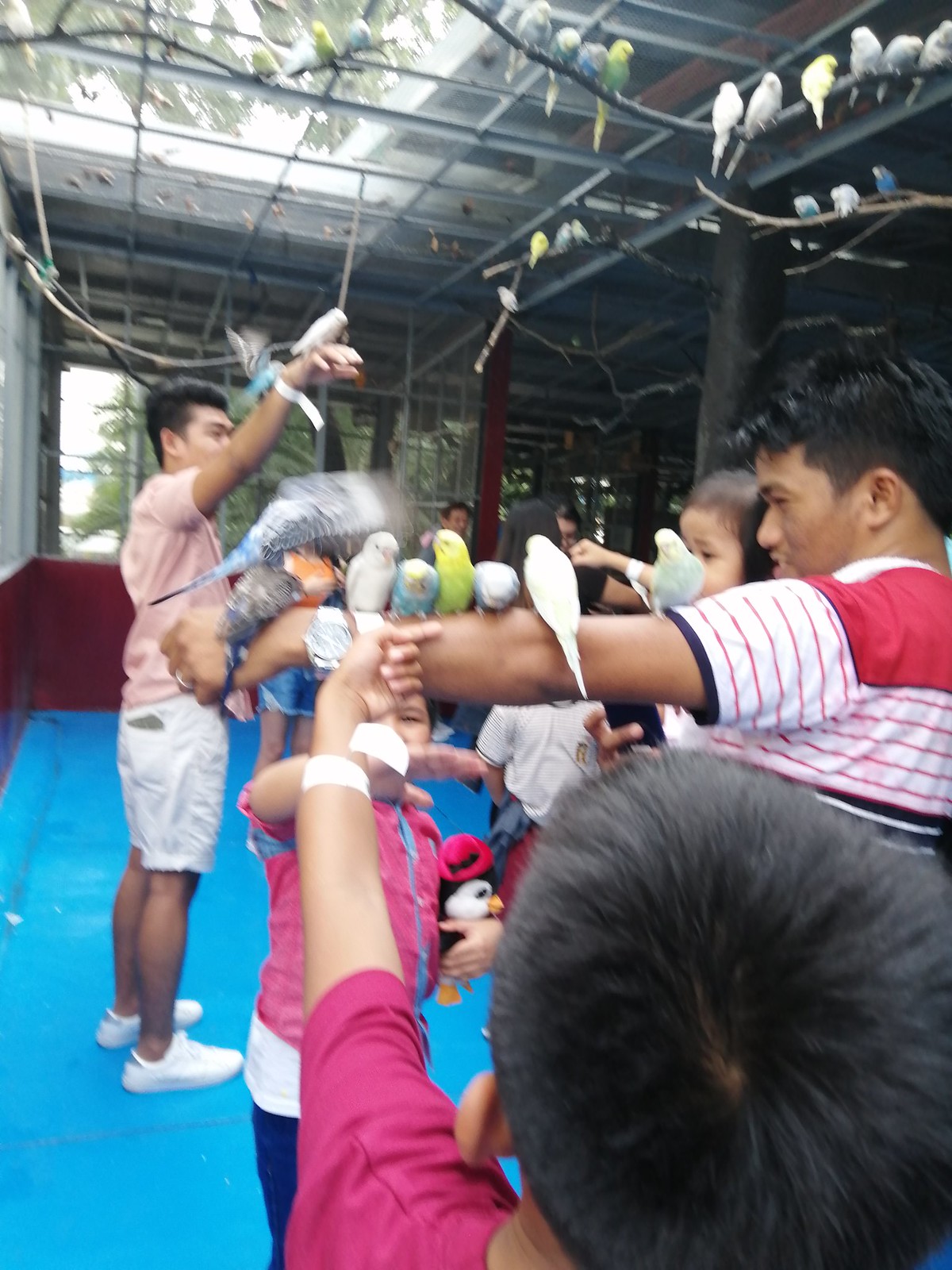In this slightly blurry photograph, a group of school-aged children is actively engaging with several colorful parakeets and other small birds in what appears to be an aviary or bird sanctuary. The aviary is spacious with a partially open ceiling that reveals a metal covering and glimpses of the sky. There is a prominent structure in the background that gives the feeling of a warehouse with a glass roof, allowing plenty of natural light to filter through. The far wall of the aviary is lined with windows, providing visibility of green trees and a distant view that resembles a beach and a body of water.

The children, excited and enthusiastic, have their arms outstretched to attract the birds. Birds of various shades—green, light blue, white, and a distinctive lime green—are perched on the children's arms. One child in the center holds a black and white stuffed penguin with an orange beak and a red hat, adding a playful element to the scene. In the top right corner, a cluster of sticks serves as perches for more birds, observing the activity below.

Two adults are central figures in the scene, guiding the children. One instructor, dressed in light shorts and a peach-colored shirt, stands with his wrist raised high, showcasing a bird to ensure all children can see. Another adult impressively holds between seven and nine birds on his arm, with one more bird attempting to land. The atmosphere is lively, with birds fluttering around and children eagerly looking for the chance to have a bird perch on them. The mix of human interaction and vibrant avian life makes this a dynamic and engaging image.